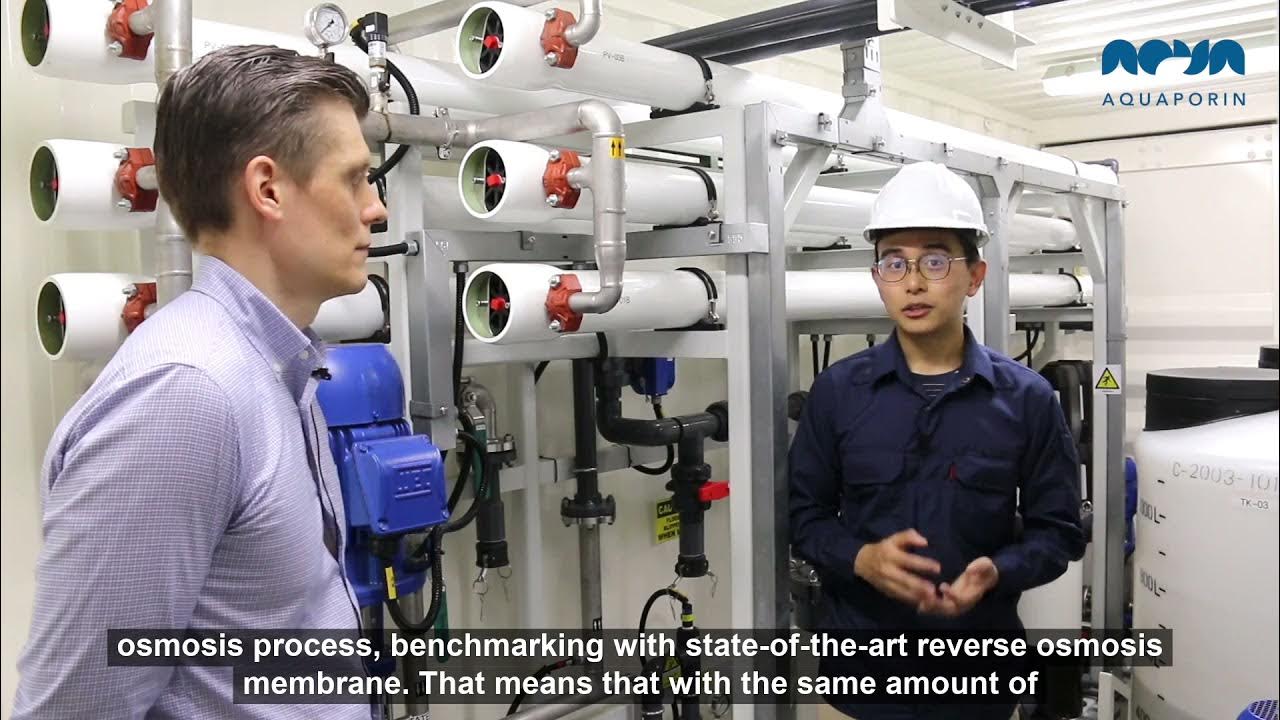The photograph depicts a scene presumably within a water treatment or power plant, showcasing two individuals amidst a complex array of machinery. On the left is a gentleman in his late 30s or early 40s with dark hair swept back, clad in a light blue-purple, fine checkered, button-down business shirt, facing to the right. He appears to be a visitor or an interviewer. Beside him, an Asian-looking technician, wearing dark-rimmed circular glasses, a white hard hat, and a dark blue-purple work outfit with front pockets, is explaining something. This technician has his hands gesturing in front of him. The background consists of numerous white tubes supported by structural elements, interspersed with red dials or tubing, in what appears to be a cramped room with whitewashed walls. A prominent poster on the right, with light blue lettering on a gray-white background, reads "Aquaporin." At the bottom of the image, against a darker background, are the words "osmosis process, benchmarking with state-of-the-art reverse osmosis membrane," indicating a focus on advanced water filtration technology.